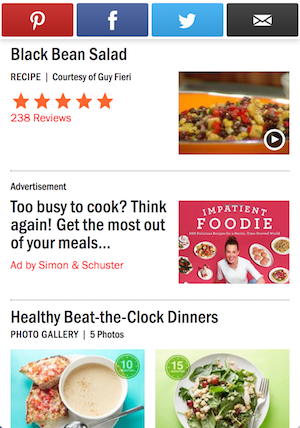The image features a variety of social media platform icons positioned at the top. The icons include a white 'P' in a red box representing Pinterest, a white 'F' in a blue box for Facebook, a light blue box with a white bird symbolizing Twitter (now known as X), and a black box with a white envelope which likely indicates email. 

Beneath these icons, the image prominently displays a recipe for a Black Bean Salad. The recipe, titled "Black Bean Salad," is credited to celebrity chef Guy Fieri. It is a five-star recipe with 238 reviews, with the stars highlighted in orange and the number of reviews in pink. The accompanying image showcases the salad in an orange dish, revealing ingredients such as black beans, corn, and onions.

Below the recipe, there is an advertisement that reads, "Too busy to cook? Think again. Get the most out of your meals." This ad is sponsored by Simon & Schuster and promotes "Inpatient Foodie." The ad features a Caucasian woman surrounded by various dishes against a pink background.

Further down, the image presents a section titled "Healthy Beat the Clock Dinners," described as a photo gallery featuring five images. Two of these images are visible. One showcases a bread or pizza-like dish with sauce and a spoon on a white plate, with a small cup containing a liquid; this is marked with the number '10' in white within a green circle, set against a blue background. The other image displays a salad featuring what appears to be feta cheese and spinach, accompanied by a fork on a round white plate. It bears the number '15' in white within a green circle, set against a very light green background.